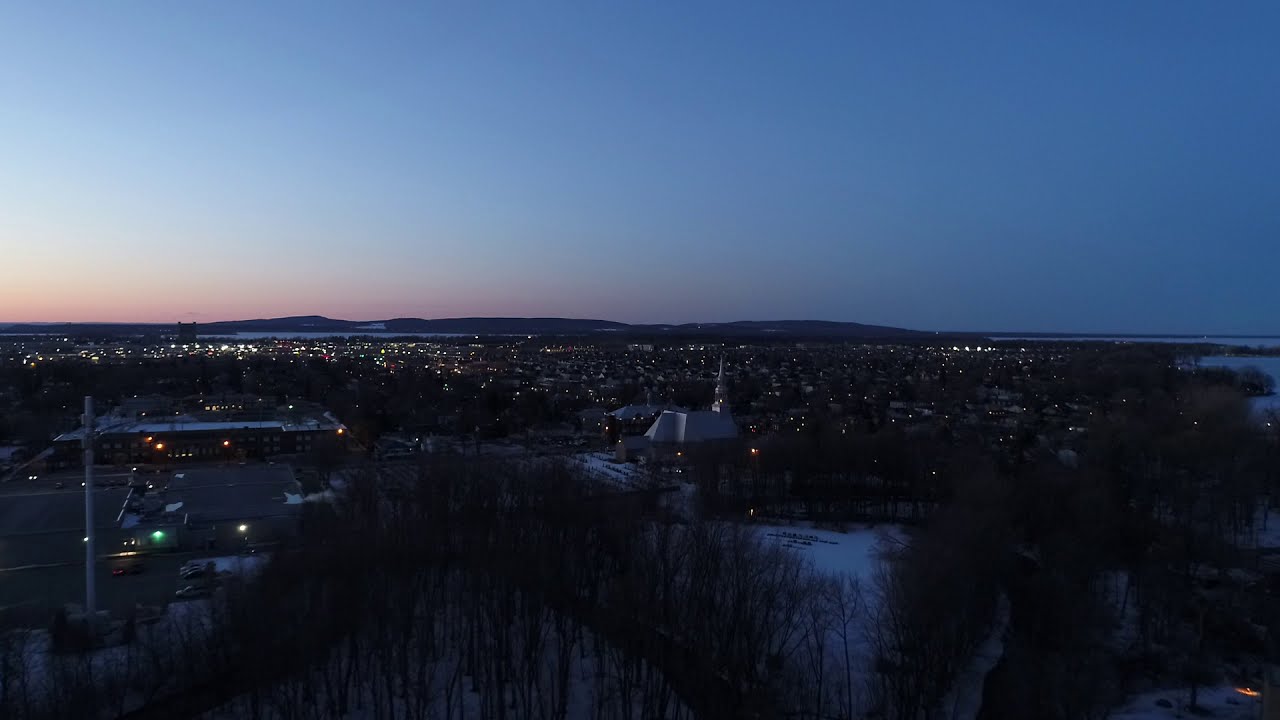The photograph, taken from a high vantage point, likely on a mountainside, captures an urban area cloaked in the gentle light of dusk or early nightfall. The sky, occupying the upper half of the image, showcases a stunning gradient transitioning from a deep blue on the right to a soft pink on the left, suggesting the recent sunset. Snow blankets the ground and rooftops, adding a serene, wintry atmosphere to the scene. In the foreground, leafless trees partially obscure the view, their branches stark against the dim light. Below, a barren parking lot with only a few cars sits on the left side of the image. The cityscape spreads out with numerous twinkling lights from small buildings and homes, indicating a peaceful, settled community. Dominating the central area of the photograph is a structure that appears to be a church, recognizable by its tall steeple, while the distant background reveals softly rolling hills. The entire scene is peaceful and calm, free of clouds and other visual disturbances.